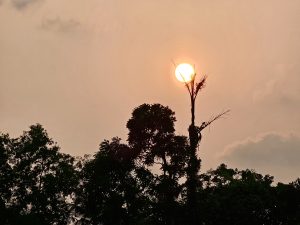The image depicts a mesmerizing scene of a tree line silhouetted against a heavily hazed sky, possibly due to pollution or a forest fire. The sun, cloaked in an intense haze, is centrally positioned behind a distinctive, tall, barren tree that resembles a palm with its fronds removed. The sky, marked by its eerie, peach-gray tone, shows shades of pink and orange radiating outward from the sun, blending into lighter hues at the periphery. Scattered dark clouds add to the atmospheric mood of the scene. Despite the turmoil implied by the haze, the setting conveys a sense of stillness and quiet beauty, as though capturing the tranquil moment of dusk descending upon a natural landscape.